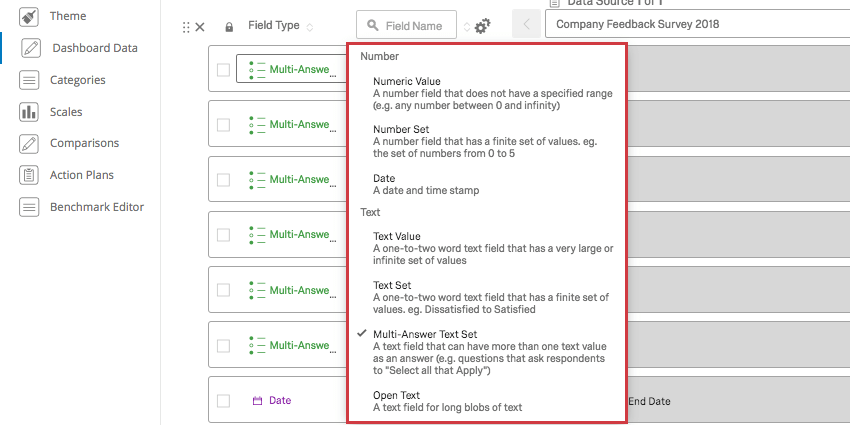This is a screenshot of a web page interface featuring various navigational and functional elements. On the left side of the image is a vertical menu with several options: "Theme," "Dashboard Data" (which is currently selected), "Categories," "Scales," "Comparisons," "Action Plans," and "Benchmark Editor." To the right, there is a panel displaying field attributes, specifically mentioning "Field Type" and "Field Name" alongside "Company Feedback Survey 2018."

Dominating the central area of the image, a red-outlined pop-up window overlays most of the background content. This pop-up window provides detailed options for different field types:
- **Number:** A numeric field without a specified range.
- **Number Set:** A numeric field constrained to a finite set of values, such as 0 to 5.
- **Date:** A date and time stamp field.
- **Text:** A brief text field that allows a very large or infinite set of values.
- **Text Set:** A brief text field with a limited set of values, for example, ranging from "dissatisfied" to "satisfied."
- **Multi-Answer Text Set:** (indicated with a checkmark) A text field permitting multiple text values as answers, ideal for questions that ask respondents to select all applicable options.
- **Open Text:** A field meant for long, descriptive text inputs.

The image orientation is landscape, being wider than it is tall, and it notably lacks any photographic content.